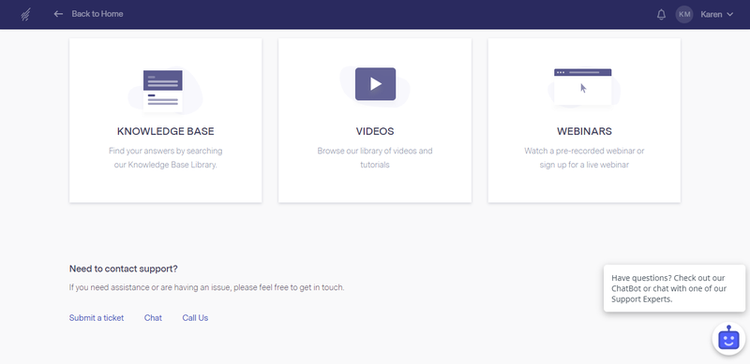The image displays a detailed user interface of a support or help center page. At the top left corner, there is a "Back to Home" button accompanied by a left-facing arrow. To the right, there is a circular icon labeled "KM" which contains a notification symbol indicating a new alert. 

Directly below that is a section titled "Knowledge Base" with the prompt: "Find your answers by searching our knowledge base library." Adjacent to this title is a screenshot of a computer displaying information, symbolized by lines representing text.

Further down, there is a section for "Videos" highlighted by a square containing a triangle, reminiscent of the YouTube logo. The description invites users to browse the library of videos and tutorials available.

Next, the "Webinars" section features a screenshot of a website with an accompanying arrow. It offers users the option to watch prerecorded webinars or sign up for live sessions.

Toward the bottom, there is a prominent section titled "Need to Contact Support?" It encourages users who need assistance or are experiencing issues to get in touch and provides three blue call-to-action buttons: "Submit a Ticket," "Chat," and "Call Us."

Finally, in the bottom right corner, there is an invitation for users with further questions to utilize the chat bot or to engage directly with one of the support experts.